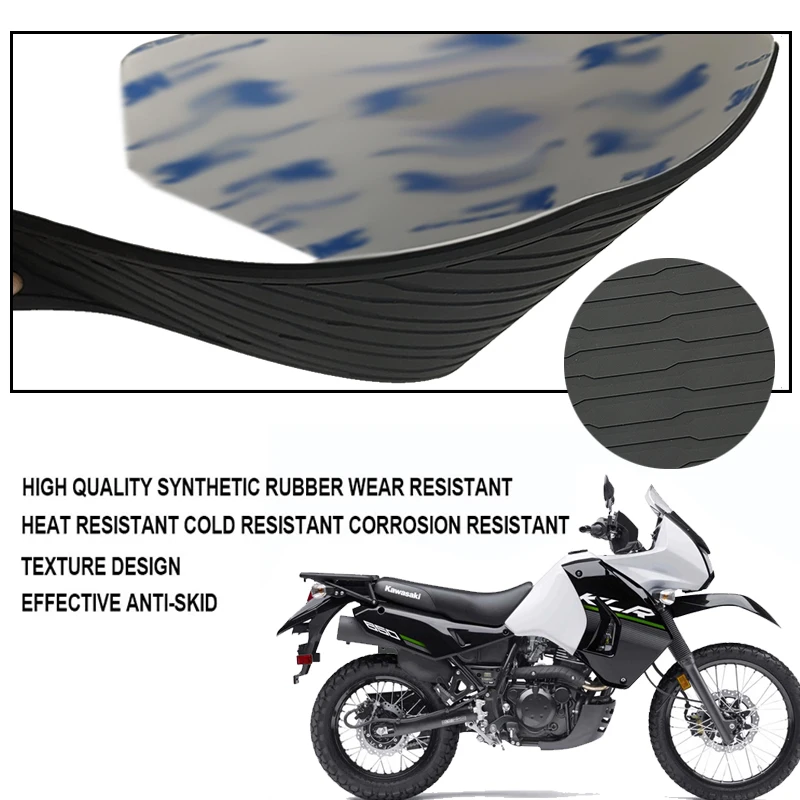This detailed image showcases a motorcycle, emphasizing its high-quality features. Positioned in the bottom right corner, the motorcycle prominently displays its leather components. To the left of the motorcycle, a list of attributes wraps around, highlighting its construction with high-quality synthetic rubber that is wear-resistant, heat-resistant, cold-resistant, corrosion-resistant, and designed with a textured pattern for effective anti-skid performance. Dominating the top half of the image is an intricate close-up view of the synthetic rubber, revealing its textured design. On the right hand side, a circular inset magnifies the rubber's detailed pattern, providing a comprehensive look at the material's superior craftsmanship and durability.